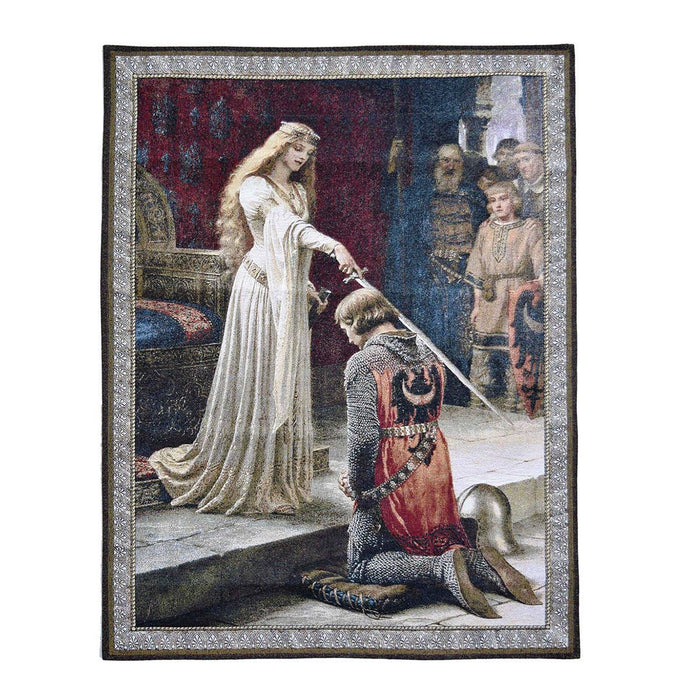The image is a detailed, color illustration set in portrait orientation, depicting a medieval knightly swearing-in ceremony. At the center of the illustration stands a princess or queen on the left side, positioned slightly back with a throne behind her. She is adorned in a long, white, flowing gown with drapey sleeves, and her long blonde hair is partially covered by a crown or headband. She gazes downward as she anoints a knight by touching his right shoulder with a sword held in her right hand. The knight, his back partially turned, kneels on a brown cushion placed at the base of a stair. He is clad in full chainmail armor covered by a red tunic displaying a black eagle emblem on the back. His silver helmet lies beside him. To the top right, several figures clad in drab-colored gowns watch the ceremony unfold. The entire scene is encased within a silver beaded frame with a brown edge, adding to the historical and artistic essence of the illustration.